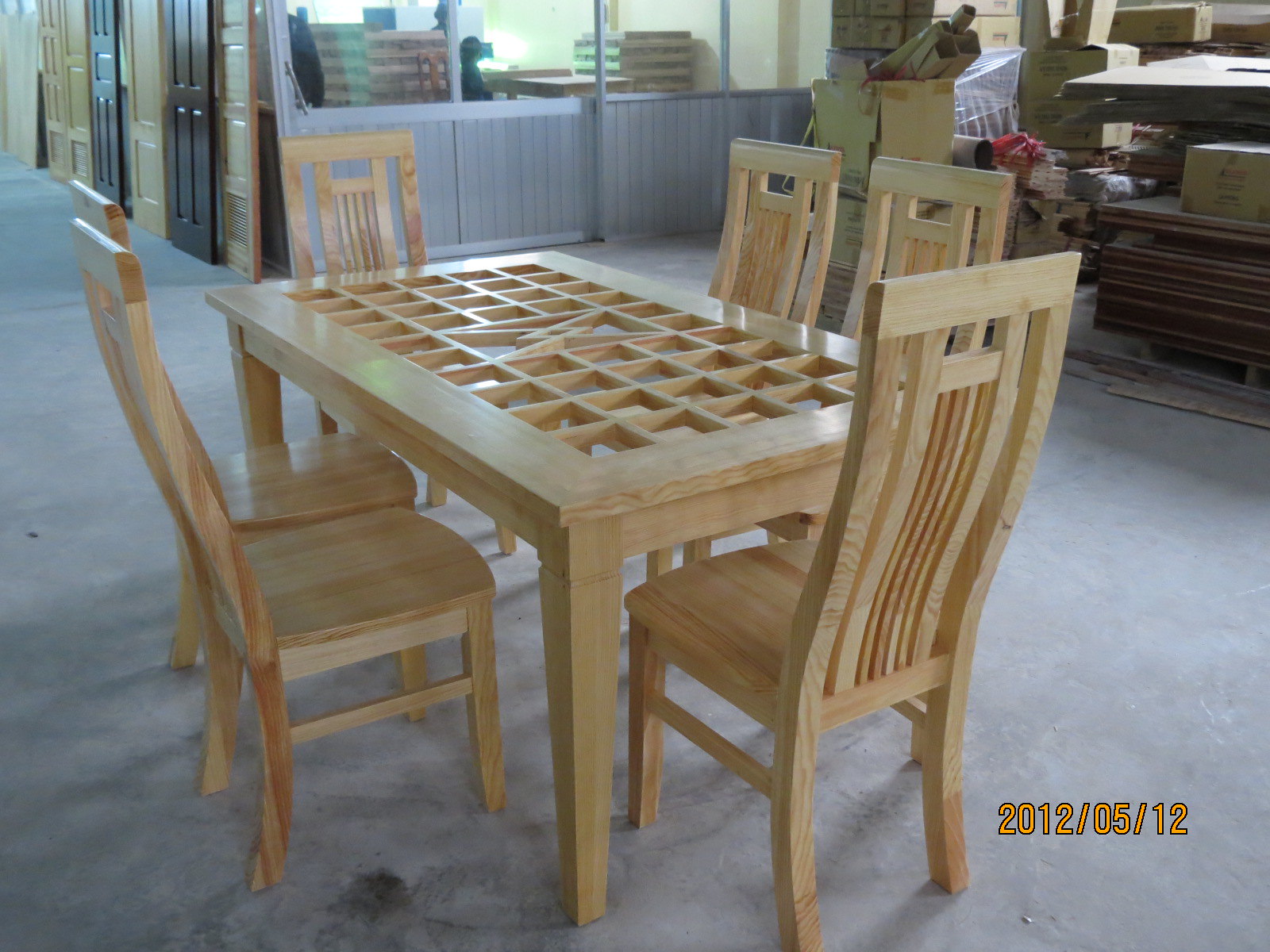The photograph depicts a dining set comprised of a light-colored wooden rectangular table and six matching chairs, situated in what appears to be an industrial woodworking workshop or warehouse. The distinctive table features an intricate lattice design in the center with multiple square and triangular cutouts, suggesting it might require additional pieces, such as glass or tiles, to make it fully functional for dining. The six chairs, arranged with two on each longer side and one at each end, share the same unfinished light wood as the table and have open-beamed backs that add to their rustic charm. The scene is bathed in a natural light that streams through tall windows, hinting at the possible presence of an office area behind glass panels. Surrounding the set, the background reveals a cluttered, industrious environment with stacks of wood, numerous wooden doors of varying hues, cardboard boxes, and crates, all resting on a dust-covered concrete floor. A date, "2012-05-12," is superimposed in orange in the bottom right corner, adding a timestamp to this compelling snapshot of a functional yet aesthetically intriguing workspace.